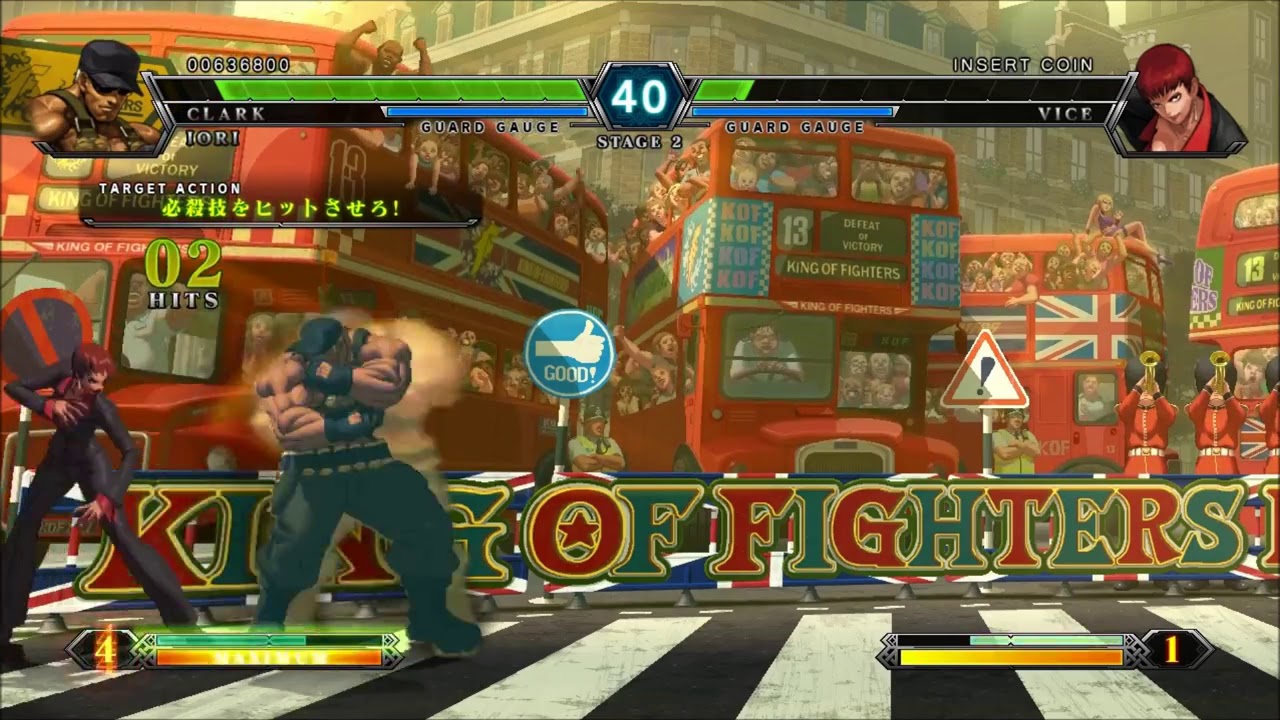This image is a detailed screenshot of a fighting game reminiscent of the classic Street Fighter style, where gameplay is limited to two-dimensional movement—forward, backward, left, and right. The scene is set against a vibrant backdrop characterized by London double-decker buses adorned with British flags. The words "King of Fighters" are prominently displayed in eye-catching red and green uppercase letters, giving the scene a lively, festive atmosphere.

In the foreground, the combat area features a distinctive black and white checkered floor. On the left side of the screen are the two fighters: the first is a heavily muscular, shirtless man named Clark, who wears dark pants, a black hat, and a black and light-colored belt. He seems poised to attack the smaller fighter next to him. The smaller fighter, named Vice, is extremely skinny with red hair and is clad entirely in a black outfit. Both characters are in dynamic fighting poses, hinting at the intensity of the battle.

At the top left corner, Clark's status information is displayed, showing his avatar, name in white letters, a green health bar, and a blue Guard Gauge bar beneath it. Similarly, on the top right corner, Vice's status is shown with her name in white text, alongside her health and guard meters. The middle of the screen features a white number "40," indicating the score or timer, with "Stage 2" written just below it.

Beyond the fighters, the background showcases bustling street scenes, complete with double-decker buses filled with cheering people and what appear to be British musicians or Queen's Guards holding yellow trumpets. This lively crowd adds to the festive and energetic atmosphere of the game. On the bottom corners, additional status areas with green and orange colors are visible, displaying a "4" on the left and a "1" on the right, possibly indicating points or lives remaining in the game.